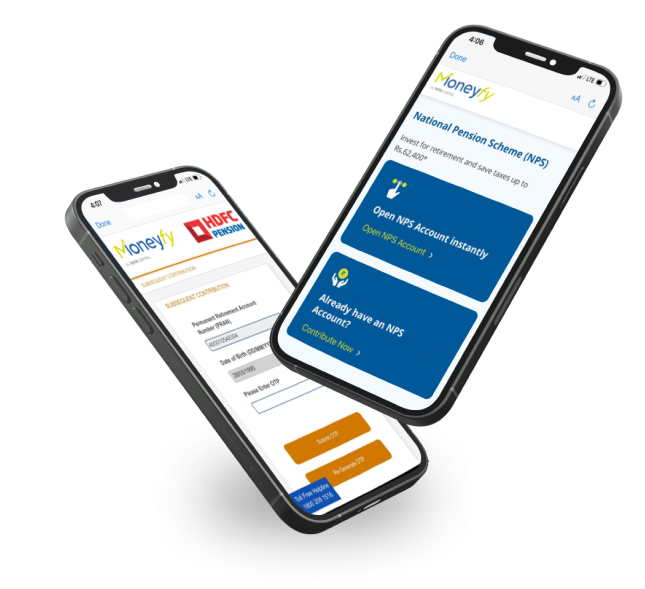The image features two smartphones positioned against a stark black backdrop. The phone on the left is displayed at an angle, leaning slightly to the left, with its screen partially visible. The display shows a white background with the text "Money FY" at the top left of the screen. The letter 'M' is colored in orange, while 'ONEY' is in blue. Following "FY," which is also in an orange shade, there's a red square containing a white square inside it. Adjacent to this is "HDFC" in black, and below that, the word "Pension" appears in blue. Below this, the rest of the screen contains a blurry message in black text that is unreadable, with two orange bars at the bottom featuring white text.

The phone on the right faces the camera more directly and leans backward toward the right side of the screen. Its display shows multiple lines of text and icons. At the top, "4, 06" appears in black text, followed by "done" in blue underneath. To the right side, there is an icon featuring a lowercase 'a' and an uppercase 'A' in blue, next to a blue refresh icon. Below this, "Money FY" is again displayed with the letter 'M' in yellow, 'ONEY' in blue, and 'FY' in yellow. The text "National Pension Scheme" (abbreviated as 'NPS' in parentheses) follows in blue. Below this, "Invest for retirement and save taxes up to RS-52400" is written in black. There is a blue box featuring a white icon of a finger pointing, with the text "Open NPS account instantly" in blue below it. Beneath this is a yellow bar that reads "Open NPS account." Further down is another blue box, this time featuring an icon of two right hands, with the text "Already have an NPS account?" in white and "Contribute now" in yellow underneath it.